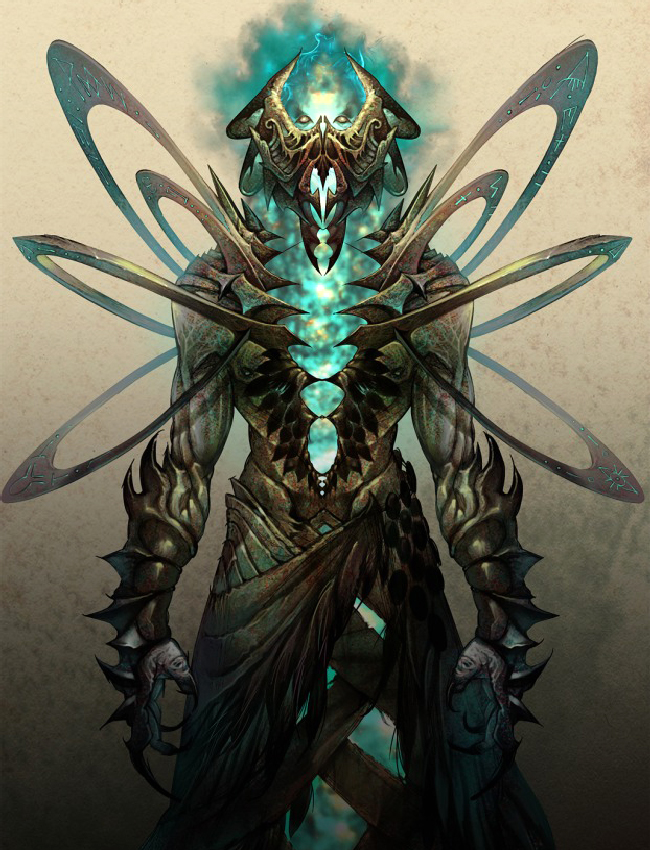This detailed graphic art or drawing showcases a fantastical creature that appears to belong to a science fiction or fantasy realm. The creature is humanoid but distinctly non-human, adorned in a taupe-colored vest-like armor that resembles a robe. Notable features include a green face with two prominent horns on either side, black eyes, and a sharp nose. The creature wears gloves embellished with spikes and has a set of blue glowing orbs running down the middle of its chest, symbolizing its dark intentions. The character also sports six wings, three on each side, shaped like upside-down U's, enhancing its otherworldly appearance. Additionally, the design includes unique shoulder pads that resemble orbital Saturn rings, further emphasizing the fantastical and sinister nature of this dark-sided character. The image is devoid of any text, focusing solely on the intricate details of the artwork.